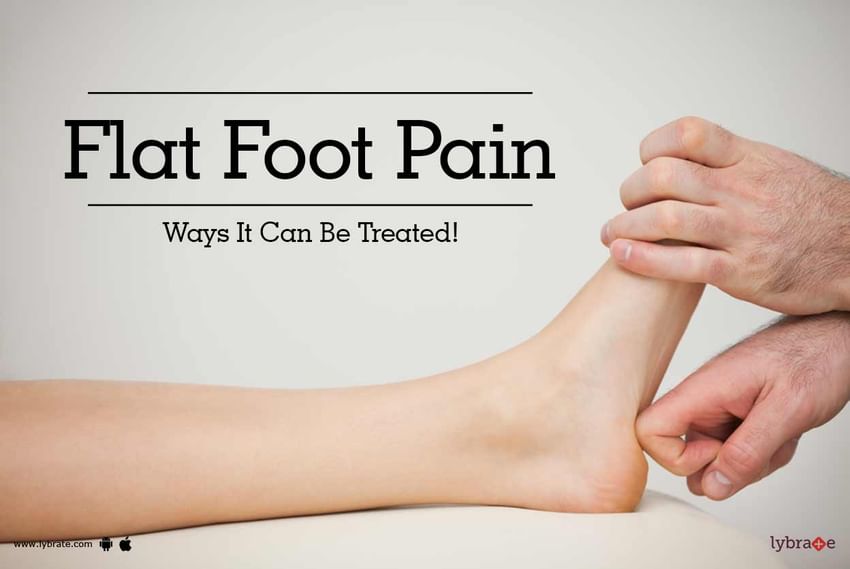The image is a detailed advertisement featuring a photograph of a leg from below the knee, stretched out horizontally. The foot is resting on a soft, light-colored cushion, possibly at the end of a bed. The focus is on a pair of very hairy hands that are actively working on the foot; one hand is gripping the toe box area while the other uses its knuckles to press into the heel. The background is a whitish-gray or light blue, providing a clean canvas that highlights the interaction. Prominently displayed in large black text on the left side of the image is the title "Flat Foot Pain, Ways It Can Be Treated." On the lower left, very small font reads "www.lybrate.com," accessible via both Samsung and Apple. On the right, the brand logo "LIBRATE" is written in purple font.